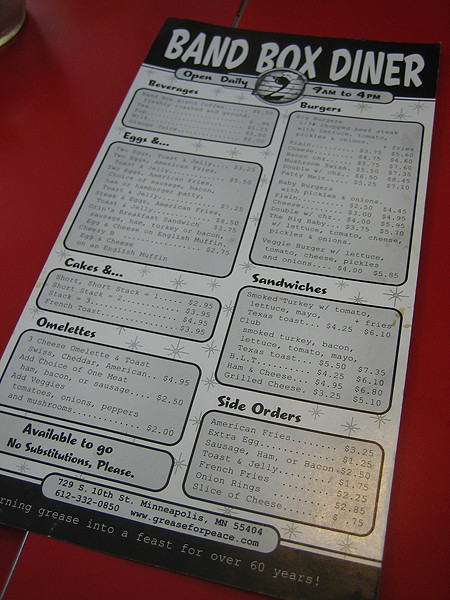This image captures a close-up view of the Band Box Diner menu, likely taken from a classic bright red table, the type typical of vintage diners. The menu occupies approximately 95% of the image, framed by a narrow border of the vibrant table. The diner operates daily from 9 AM to 4 PM.

On the left side of the menu, the offerings are divided into several sections. At the top are beverages, followed by a section titled "Eggs and..." which lists various egg dishes and accompanying items. Below that is "Cakes and..." likely detailing dessert options. Underneath, there is a variety of omelettes available. A note at the bottom of this section states, "Available to go. No substitutions please."

The right side of the menu features burgers at the top, followed by a variety of sandwiches, and then side orders. At the very bottom, the diner’s slogan reads, "Grease into a Feast for Over 60 Years," though the word "burning" is obscured, suggesting the full slogan might be "Burning Grease into a Feast for Over 60 Years."